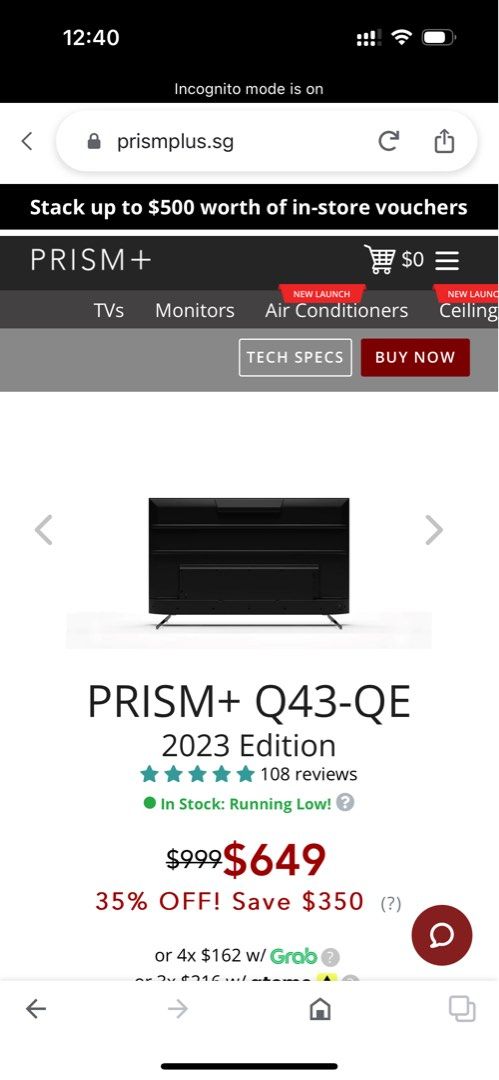The image shows a mobile device screen displaying a website. The time displayed at the top is 12:40, with signal indicators showing three out of four bars for data and three out of three bars for Wi-Fi. The battery icon in the upper right-hand corner shows approximately 75% charge. The top section indicates that incognito mode is active, as noted in white text.

Below this, in the main portion of the screen, is a search bar featuring the URL "prismplus.sg" along with a refresh/upload-download icon. Directly underneath, in a black header with white text, the website advertises: "Stack up to $500 worth of in-store vouchers." Next to this text is a shopping cart icon showing a "$0" balance.

The website navigation includes links for "TVs," "Monitors," and "Air Conditioners," each marked with "New Launch." Additional options include "Tech Specs" and a prominent red "Buy Now" button.

An image of a sleek flat-screen television, labeled "Prism+ Q43QE 2023 Edition," is prominently featured. The TV has a five-star rating based on 108 reviews and is listed as "In Stock" with a note that availability is "Running Low." The original price of $999 has been slashed to $649, reflecting a 35% discount and a savings of $350.